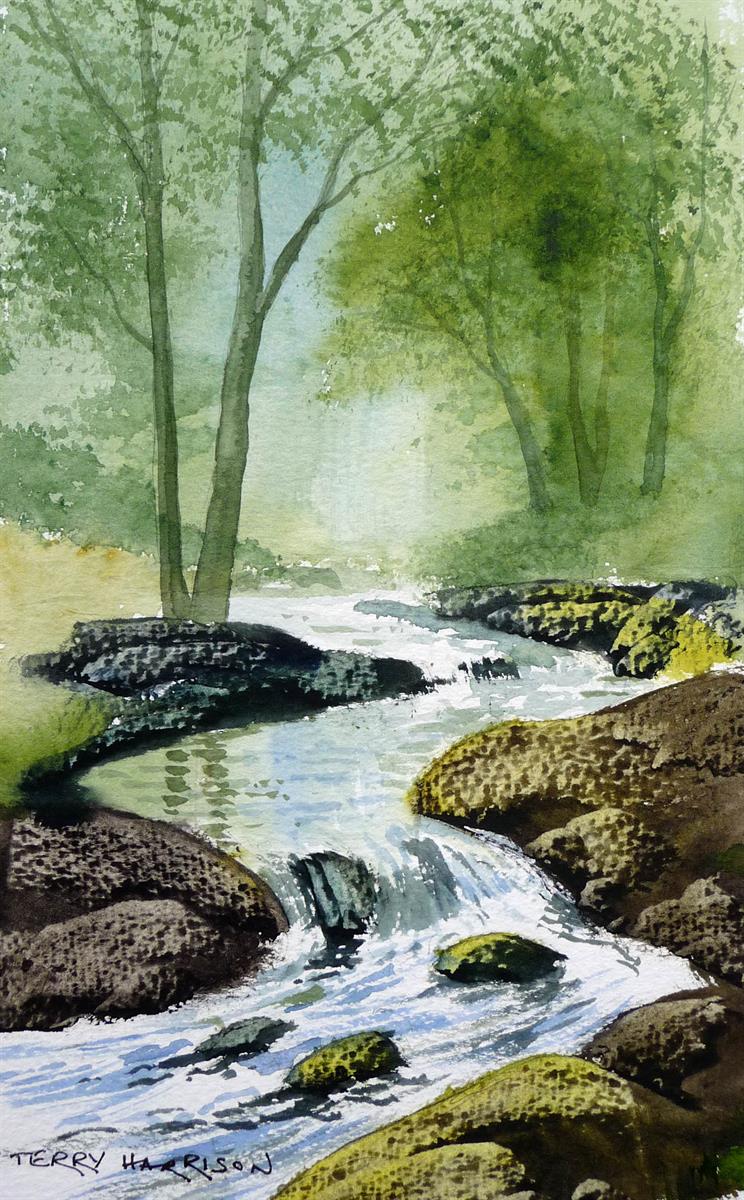This is a detailed watercolor or mixed-media painting of an outdoor forest scene featuring a winding river. The painting, titled by Terry Harrison, is taller than it is wide. Dominating the background are deciduous trees with visible trunks, branches, and green leaves creating a canopy effect. Beneath the trees, low-lying brush and green bushes add to the lush appearance. 

The river, flowing from the center, first curves to the left, then right, continuing this winding pattern until it exits in the bottom left corner. It is depicted in varying shades of blue and green, reflecting the surrounding trees. Along its course, the river cascades over multiple rock outcroppings, including a small slope forming a modest waterfall. The water below the waterfall turns frothy and white with streaks of dark blue. There are moss and algae-covered rocks both in the river and near its edges, with three noticeable boulders in the middle of the stream.

The rocks on the left side of the river are primarily brown and beige, progressing from dark blue almost black near the waterfall to yellowish-green hues further downstream. On the right side, the rocks display a mix of brown and yellow tones. The banks are varied too, with grass and a low bank on the right under the trees completing the scene, while a clearing with brown and beige hues appears on the left. Overall, the painting's intricate details and color variations create a serene and dynamic representation of a forest river scene.